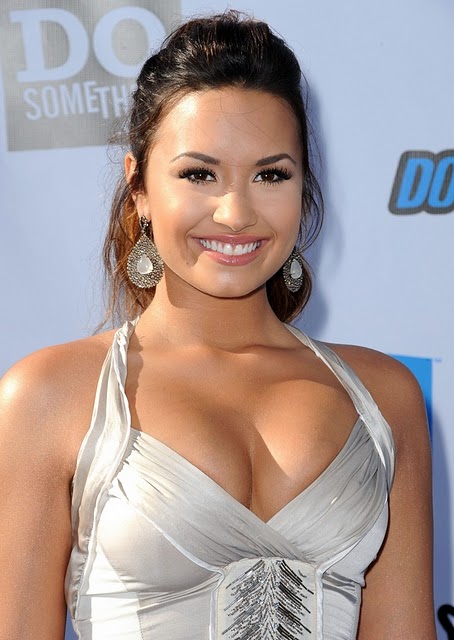The image features Demi Lovato standing confidently in front of a light blue backdrop that prominently displays the phrase "Do Something" within a rectangle. Lovato is positioned at a slight angle, looking off to her left, with a radiant smile that reveals her teeth. She is wearing a white dress with halter straps that emphasize the openness of the top, showcasing her cleavage. The dress features a distinctive black patterned design running down the center below her bust. Her hair is styled in a sleek updo, pulled back at the base with the top combed back. She accessorizes with elegant pear-shaped earrings, each featuring a smaller pear-shaped accent. The image is brightly lit, likely taken in natural light at an outdoor event, and the overall clarity is high, highlighting Demi Lovato's beauty and stylish appearance.